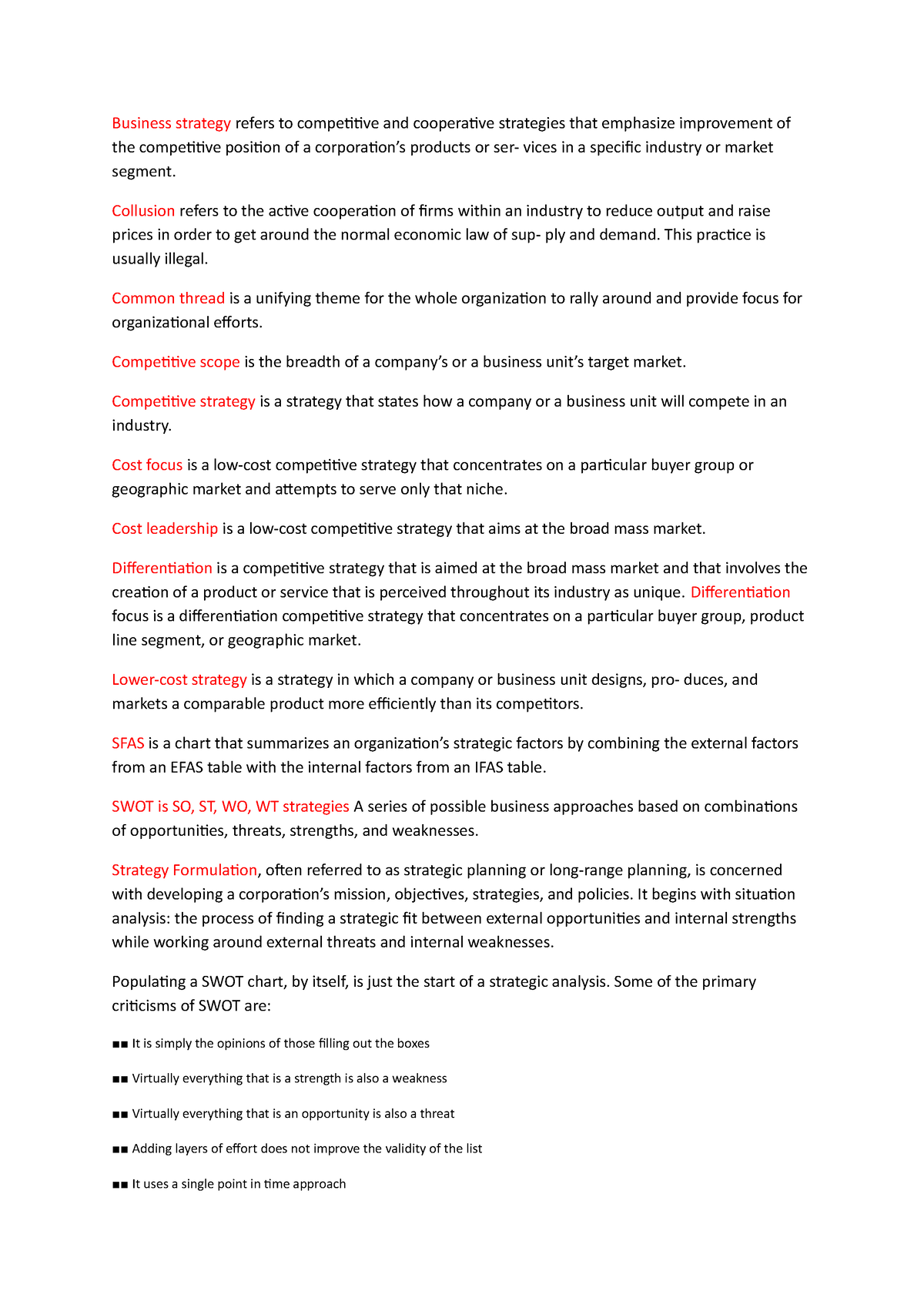In the photograph, there is an article featuring a visually striking layout with white, red, and black colors. The central focus of the article is "Business Strategy" prominently displayed in red text. This term is defined as the competitive and cooperative strategies that aim to enhance the competitive position of a corporation’s products or services within a specific industry or market segment.

Highlighted in red, several key concepts are explained in detail:

- **Collusion**: Defined as the active cooperation of firms within an industry to reduce output and manipulate prices, circumventing the normal economic laws of supply and demand. This practice is typically illegal.
  
- **Common Thread**: Identified as a unifying theme that underlies and rallies the entire organization, providing a focal point for collective efforts.

- **Competitive Scope**: Described as the breadth of a company’s or business unit’s target market.

- **Competitive Strategy**: A strategy outlining how a company or business unit will compete within an industry.

- **Cost Focus**: A low-cost competitive strategy that targets a specific buyer group or geographic market, aiming to serve only that particular niche.

- **Cost Leadership**: Another essential term highlighted in red, though lacking a specific definition in the given context, suggests a strategy focused on being the lowest cost producer in an industry.

The detailed layout of the article suggests a comprehensive examination of business strategies with a clear focus on how companies can navigate competitive environments.